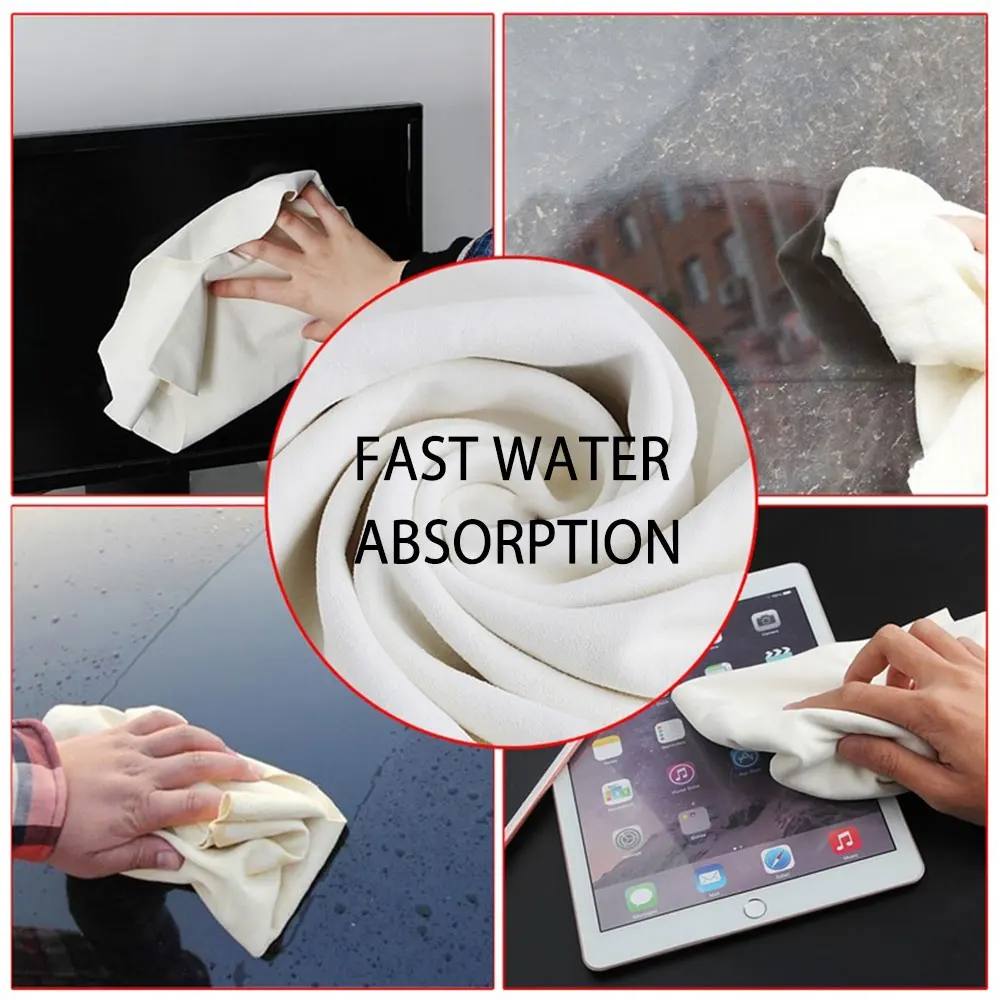This promotional image features a highly absorbent white rag, designed for versatile cleaning tasks. The layout consists of four square photos arranged in a grid, with a central circle overlapping each corner. At the center, the twisted up rag is displayed with the bold text "Fast Water Absorption" in black. Each of the four surrounding images demonstrates the rag being used to clean different surfaces: the upper left shows someone wiping a computer monitor, the upper right depicts the rag cleaning a dirty window, the lower left illustrates it being used on a car window, and the lower right features it cleaning a tablet screen. The white, creamy rag promises quick and effective water absorption, making it ideal for making various glass and screen surfaces shiny and clean.